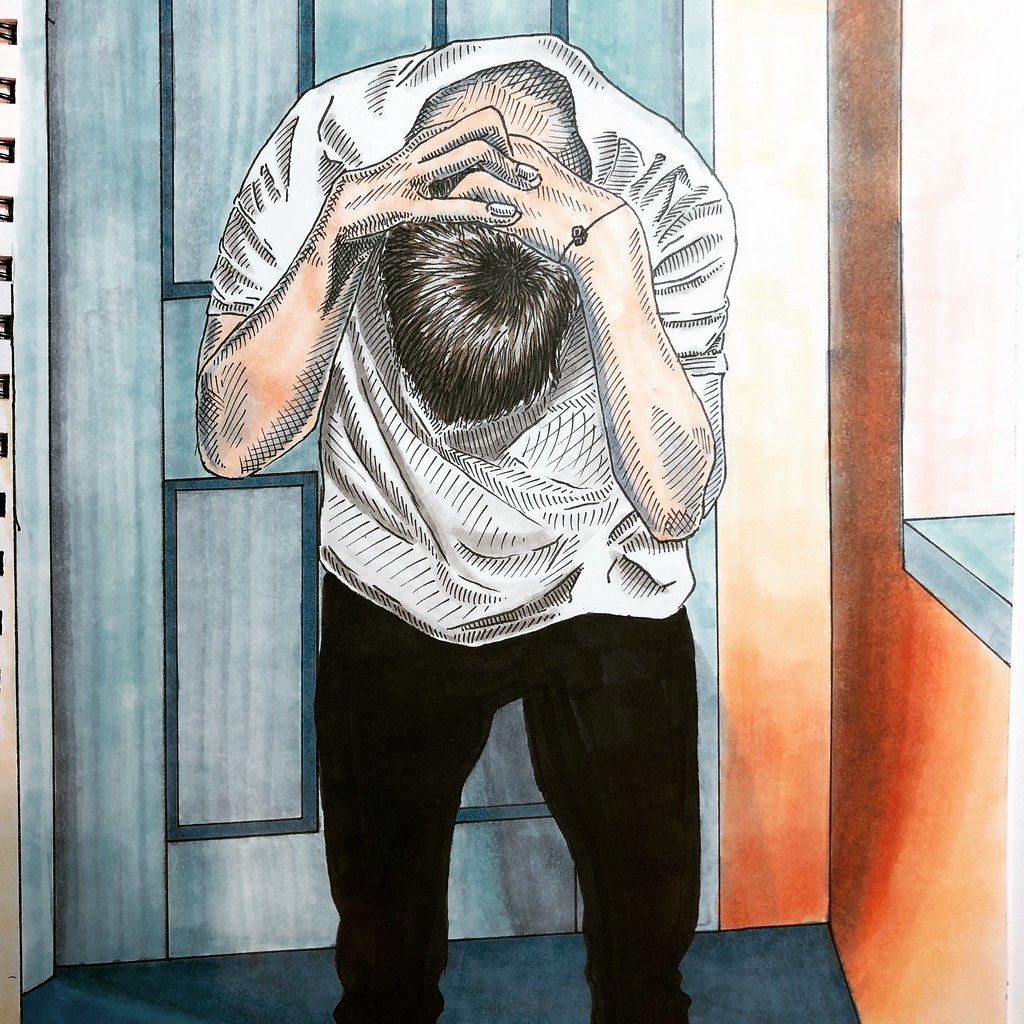This detailed, hand-drawn sketch, rendered in pen or pencil, features an androgynous figure posed in a gesture of intense emotion or contemplation. The figure's hands clasp their neck, and they bow forward, as if weighed down by a heavy burden or lost in deep thought. They wear a simple white top with short sleeves, paired with black pants, which emphasize the soft, sketchy lines of the drawing. The setting is a sparsely furnished room, with a distinctive light blue door framed by green trim serving as a subtle yet colorful backdrop to the poignantly illustrated scene.